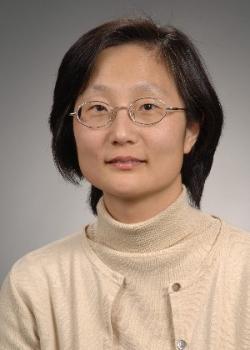This is a detailed portrait photo of an Asian woman with black, shoulder-length hair that is parted at the forehead. She is seated in front of a gradient gray wall that transitions from dark at the top to light at the bottom. The image captures her head and a portion of her upper body, focusing on her face and shoulders. She is wearing circular eyeglasses and has a calm, pleasant expression with a slight smile. Her attire consists of a camel beige outfit, featuring a base layer of a beige turtleneck and an open cardigan of a similar color. The cardigan includes buttons along the front. Her overall appearance is professional, suggesting she might be a professor or a doctor.